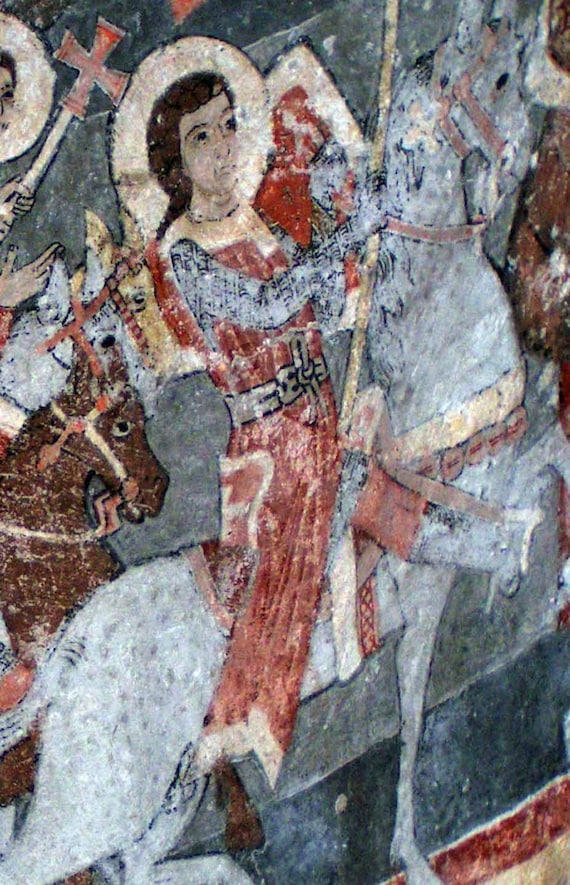This image is a close-up photograph of a detailed mural, likely depicting a historical or religious event, with dominant colors being vibrant reds, deep blues, shades of brown, and muted grays. Central to the mural is a figure, possibly St. George, that's riding a white or silver horse speckled with black spots, its head lifted towards the upper right corner. The figure, dressed in a red robe with white sleeves and wearing a tan hat, has long brown hair and is shown with a white halo, indicating sainthood. The saint holds a staff, possibly a religious symbol with a cross at the end. The horse is accentuated with gray boots in the stirrups of a cloth-like saddle. Surrounding the central figure are other horses, primarily in brown and silver hues, likely ridden by knights. One of these knights is holding another staff with a cross, a common symbol of the Crusades. In the top left corner, another haloed figure's partial face and hat can be seen, bringing a sense of depth and mystique. The background features a dark gray color with a subtle pattern of gray, red, and tan stripes, enhancing the mural's historical and almost medieval essence.